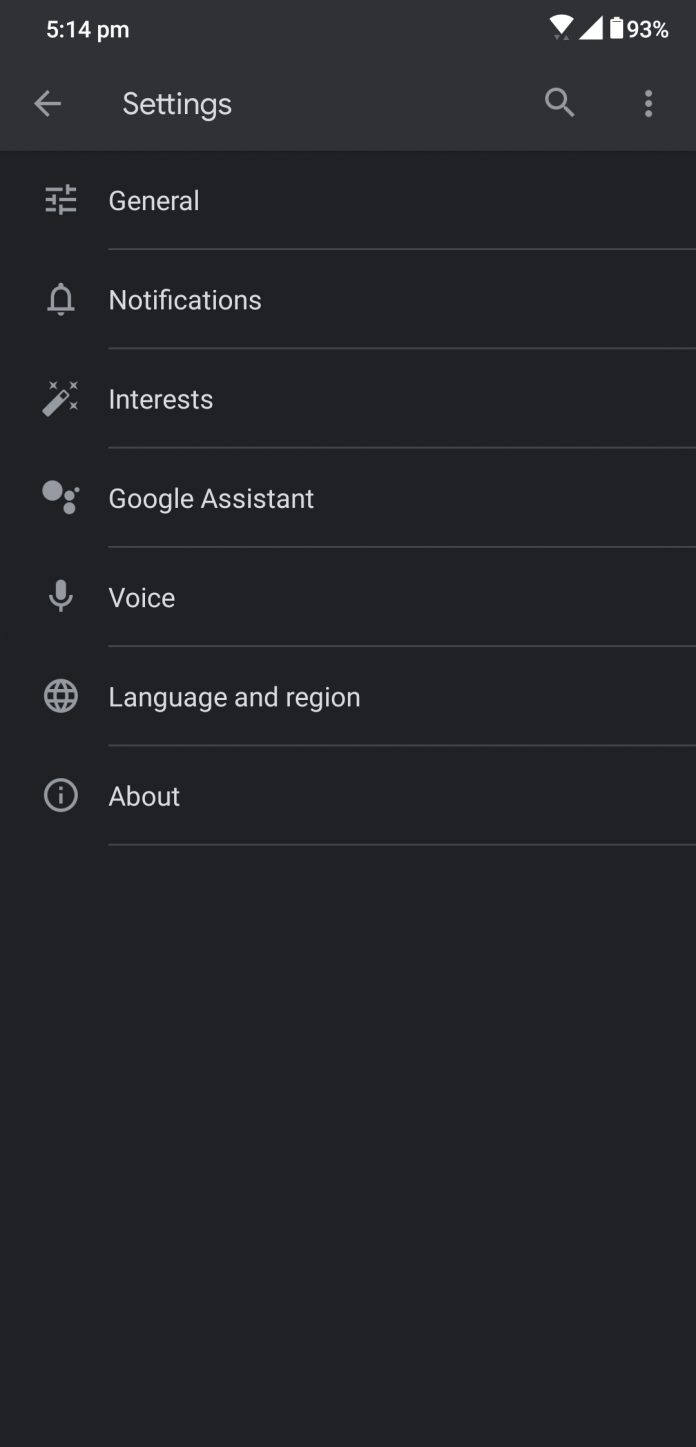A smartphone screen displays the Settings menu in stark contrast, with a black background and white text. The status bar at the top shows the time as 5:14 p.m. on the left, with Wi-Fi signal strength and a battery level of 93% on the right. The Settings menu lists various options: General, Notifications, Interests, Google Assistant, Voice, Language & Region, and About.